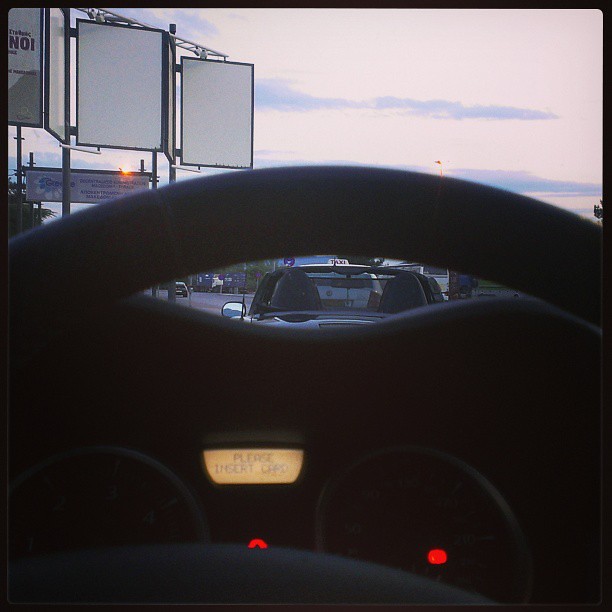This photograph, taken from the driver's seat of a dark interior car, focuses on the steering wheel and the center dashboard in the dimly-lit cabin. Prominently displayed on the dashboard is a small screen with the message "Please insert card," suggesting it might be a taxi. Through the steering wheel's opening, the image captures the view of the road ahead. Driving behind several vehicles, including a convertible and a taxi, the scene hints at a possible traffic jam. The sky, tinged with hues of pink, blue, and white, suggests the time is either sunrise or sunset. To the top left corner of the image, large, nearly rectangular white signs with multiple panels are visible, alongside some red lights, adding to the bustling yet serene atmosphere of the shot.